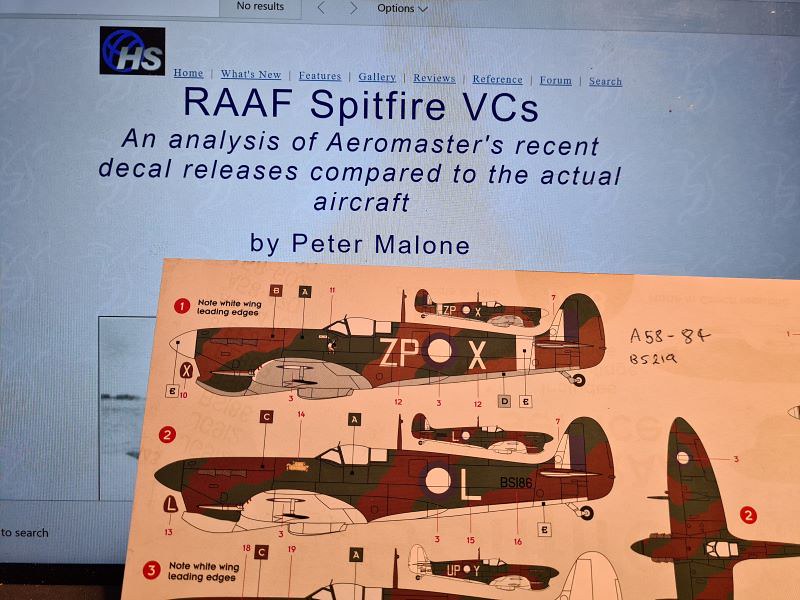The photograph captures a computer screen displaying a detailed webpage about the Royal Army Air Force Spitfire VCs, specifically an analysis by Peter Malone of AeroMaster's recent decal releases compared to the actual aircraft. The screen shows a series of drawings depicting various World War II aircraft in different perspectives, including side and top views, with each diagram labeled with lettered and numbered notes pointing to different parts of the planes. The left profile of the aircraft is prominently annotated, and there’s a photograph partially obscured by an orange paper card propped against the screen. Handwritten on this card are the numbers "A58-84" and "B5219". At the top of the webpage, several navigation options are visible, including items, what's new, features, gallery, reviews, reference, forum, and search, aligned horizontally. Additionally, the top left corner of the screen features a black box with a blue and gray logo containing white text "HS" and a globe image. The image highlights the intricacy in the comparison of decal placements on the aircraft, captured against the backdrop of a webpage, merging both digital and physical representations of historical aviation analysis.